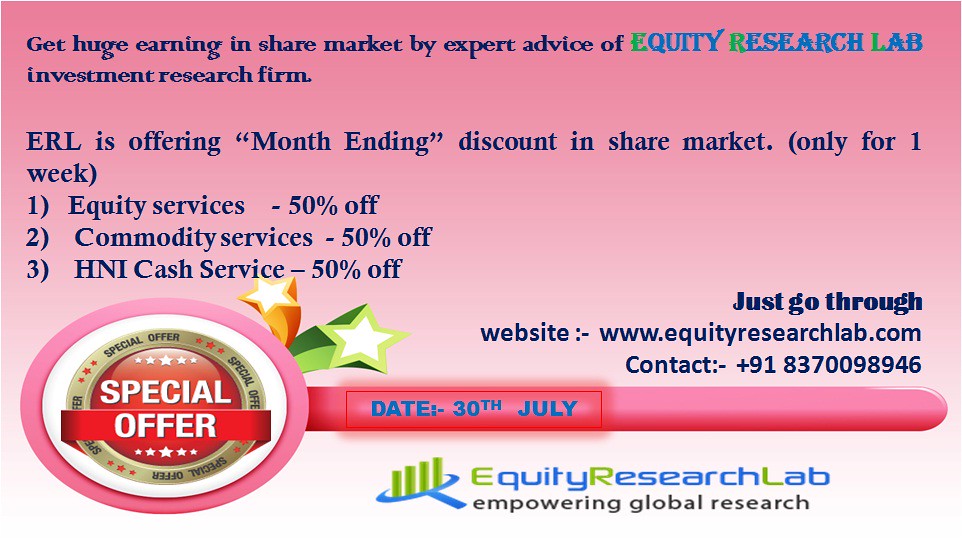This advertisement features a prominent gradient background that transitions from dark pink at the top to bright white at the bottom. At the top of the image, in bold blue text, the ad reads: "Get huge earnings in the share market by expert advice of Equity Research Lab, an investment research firm." Notably, "Equity Research Lab" is written in larger blue letters with the initials "E", "R", and "L" highlighted in green. The ad promotes a special month-end discount valid for one week, offering up to 50% off on three types of services: 1) Equity Services, 2) Commodity Services, and 3) HNI Cash Services. 

The advertisement advises viewers to visit their website at www.equityresearchlab.com for more details and provides a contact number in the bottom left corner: +918370098946. A distinctive "Special Offer" logo is also featured in the bottom left corner, with "Special Offer" written in red with white letters, encircled by a gold border. To the right of this logo, the date "30th July" appears in blue text. Just below this date, "Equity Research Lab" is reiterated in blue and green text, along with the tagline "Empowering Global Research."

Overall, this detailed advertisement blends striking colors with clear, bold text to promote limited-time discounts on investment services provided by Equity Research Lab.